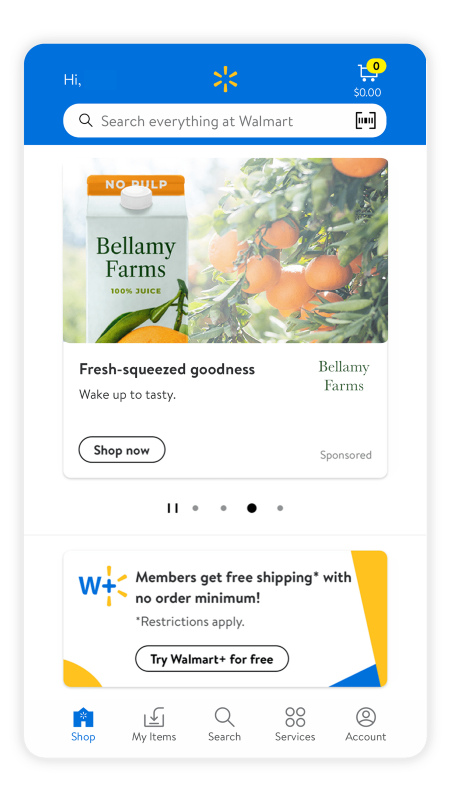The screenshot captures the user interface of the Walmart Plus or Walmart Groceries app on a smartphone. The top of the screen prominently features the Walmart logo, a yellow spark with lines radiating from a central dot, and a greeting message that simply says "Hi".

On the right side of the screen, there's an empty shopping cart icon with a counter showing zero items. Below this area, there's a search bar labeled "Search at Walmart", accompanied by an alternative option to use a scanner button. This feature allows users to scan product barcodes with their phone for easier searching within the app.

The central part of the screen displays an image advertisement for "Bellamy Farms 100% Juice No Pulp." The carton is showcased with the brand name, Bellamy Farms, written in green, alongside an image of an orange with a stem. To the right of the carton, there is a vivid picture of oranges growing on a tree. The promotional text reads "Fresh Squeezed Goodness, Wake Up to Tasty," emphasizing the juice's freshness. Further, there's a "Shop Now" button in a circular icon on the left side, and a "Sponsored" label in gray on the right.

The app is currently showing the third out of four slides in a rotating slideshow of promotional images. Below the slideshow, there's a box stating, "Members get free shipping" with an asterisk denoting an order minimum, followed by a prompt to "Try Walmart for free."

At the bottom of the screen, the navigation bar provides options to "Shop" (highlighted in blue), access "My Items", conduct a "Search", check available "Services", and manage "Account Information".